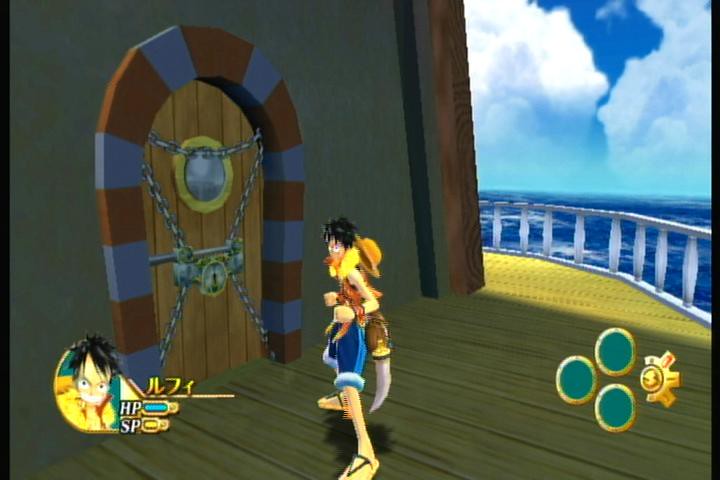The image depicts a cartoon scene set on the wooden deck of a ship, showcasing a central structure made of rough-hewn planks. Dominating this structure is an imposing wooden door, intricately wrapped in chains and secured with multiple locks, including a large, old-fashioned keyhole. The door features a round porthole and is bordered by stripes in shades of purple and brown that draw the eye inward. 

In the middle of the scene stands a Muppet-like character, sporting a pair of sandals, rolled-up blue-jean shorts, and a backpack equipped with at least one knife. The character also wears a hat, enhancing his adventurous appearance. Notably, an additional picture of this animated figure is situated in the bottom left corner of the image, hinting that this scene might be from a video game.